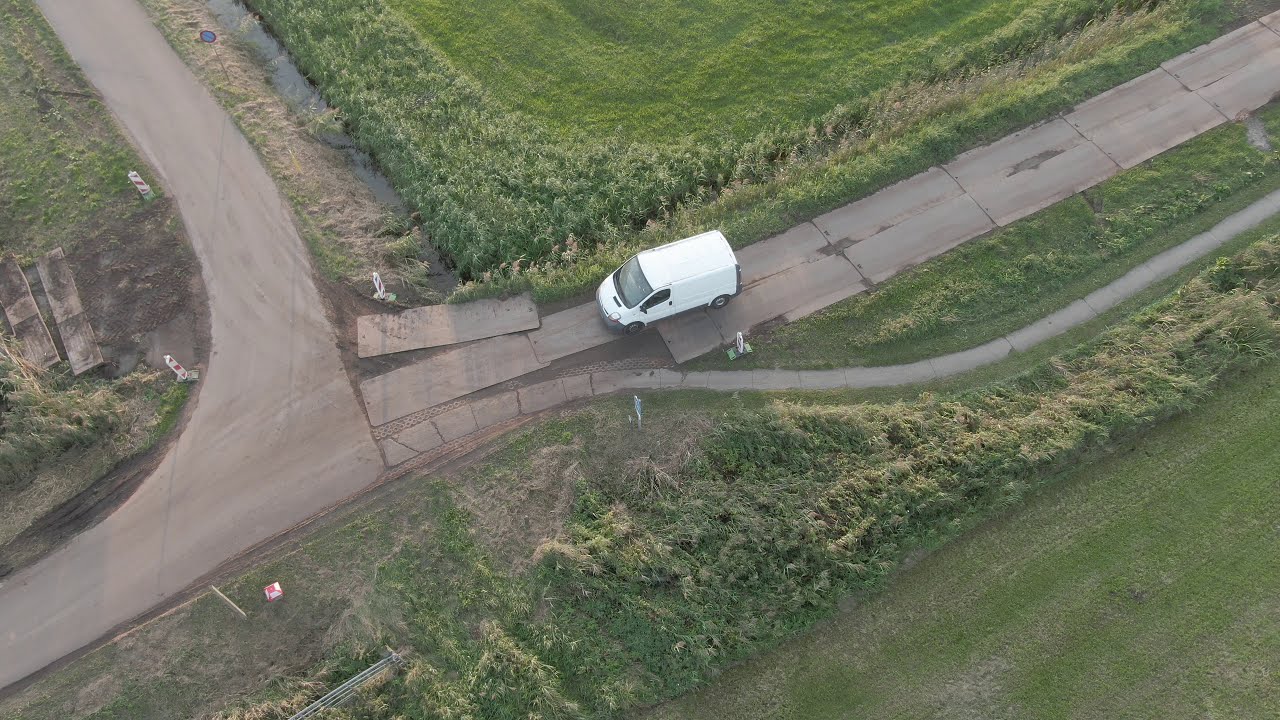This horizontally aligned rectangular aerial photograph, taken during the daytime, showcases a rural landscape with intersecting roads and green fields. The upper portion of the image features a grassy field bordered by trees. Below this, an older, single-lane road made of rectangular concrete pieces stretches diagonally from the lower left to the upper right. This road appears rough and broken, with some concrete pieces displaced to the side. A white minivan with its headlights on is prominently situated in the center of the image on this road. Adjacent to the older road, a narrow pathway or walkway extends and slopes downwards. In the upper left-hand side, a more well-maintained solid concrete road runs parallel, showing no visible cracks. At the bottom of the image, another lush green field is bordered by a row of trees, encapsulating the serene and rustic essence of this aerial view.